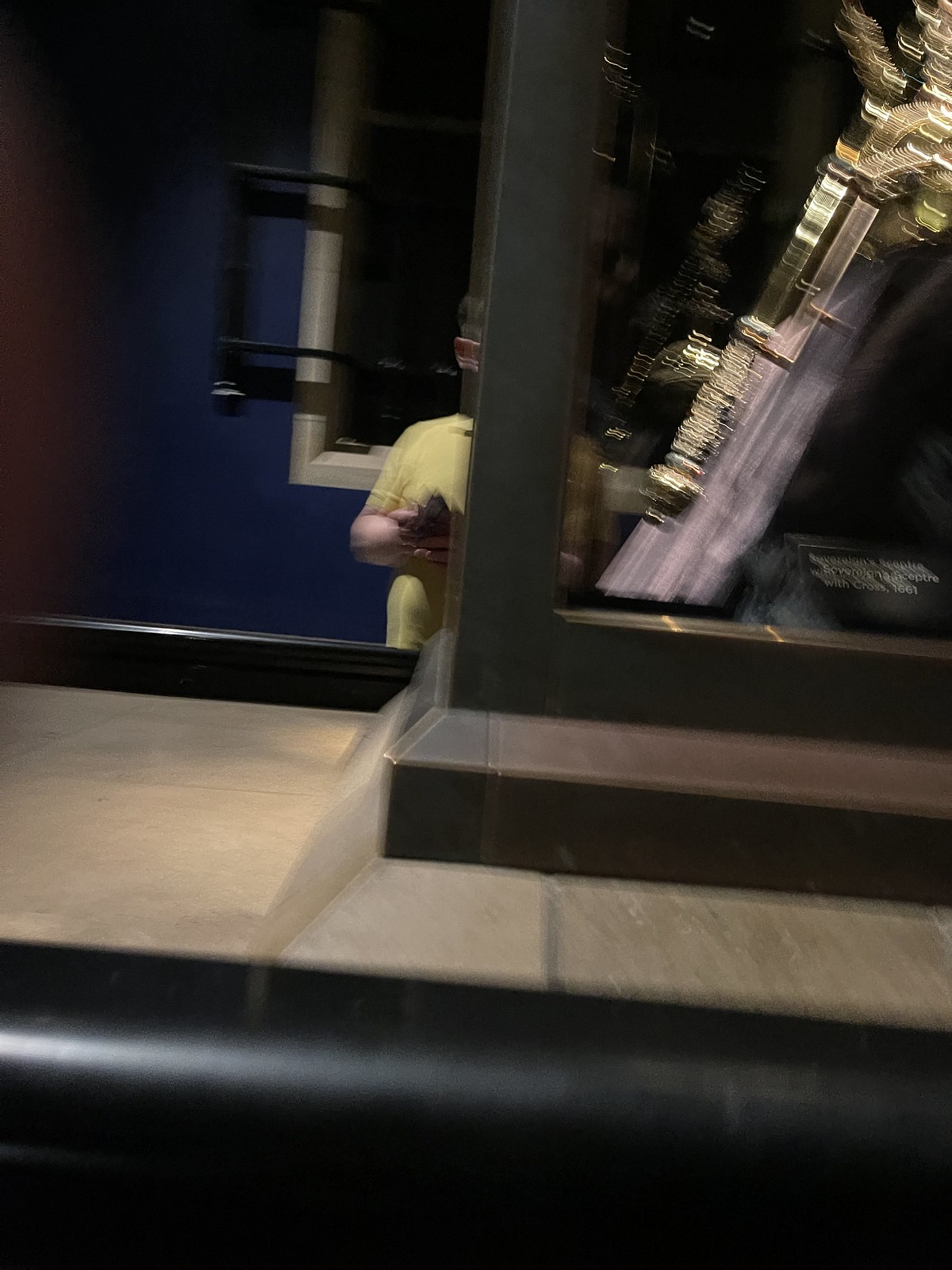In this dimly-lit photograph taken inside what appears to be a museum, a person is prominently but partially visible, standing just behind a black pole or column. The individual, whose facial features are obscured by the post, wears a short-sleeve, straw-colored yellow shirt. The person is holding an indistinct object in their right hand, and their left side is the only part clearly visible. The image appears slightly blurry, adding to the difficulty in identifying the object this person is holding. The background reveals a dark navy blue or royal blue wall with a stone-outlined window and an exhibit display nearby featuring imitation stone tiles or large, light brown marble tiles. Reflections in the display's glass and a label with three lines of text, including something resembling "width cross 1661" can be seen. The display itself, possibly showing an animal habitat with elements like a tree, contributes to the museum-like ambiance of the setting.